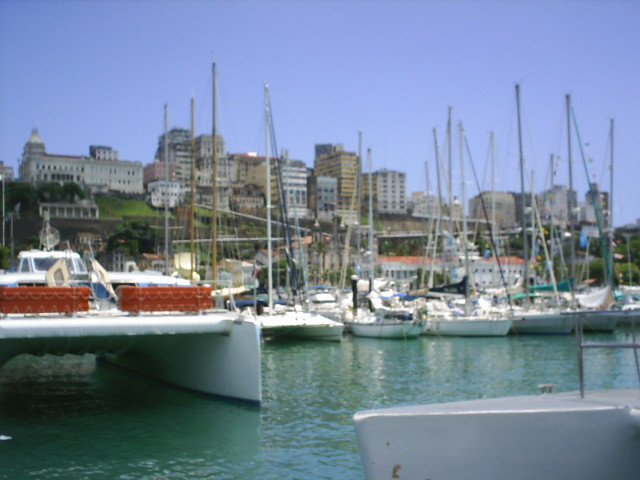The image captures a vibrant marina scene set against a backdrop of a bustling city. Clustered tightly together, numerous white sailboats, with their tall masts standing bare of sails, fill the foreground. These boats are docked in a compact fashion, creating a dense and busy atmosphere. To the left, a distinctive catamaran stands out among the regular sailboats, accompanied by another catamaran nearby and possibly a third one further to the right, adding variety to the otherwise uniform collection of vessels.

In the front of the image, a silver-gray dock is visible, equipped with fixtures for mooring boats. The water in the marina glistens with a greenish-blue hue, adding to the image's lively color palette. On the left side of the dock, there appear to be red benches or storage containers, though it's difficult to discern their exact purpose.

Behind the marina, a cluster of city buildings rises up the hillside, their multi-story structures crowned by a clear, bright blue sky that suggests a sunny day. The slope features patches of green grass, enhancing the scene's natural beauty and contrasting with the urban elements. The overall composition paints a picture of a serene yet dynamic coastal cityscape, bustling with nautical activity.